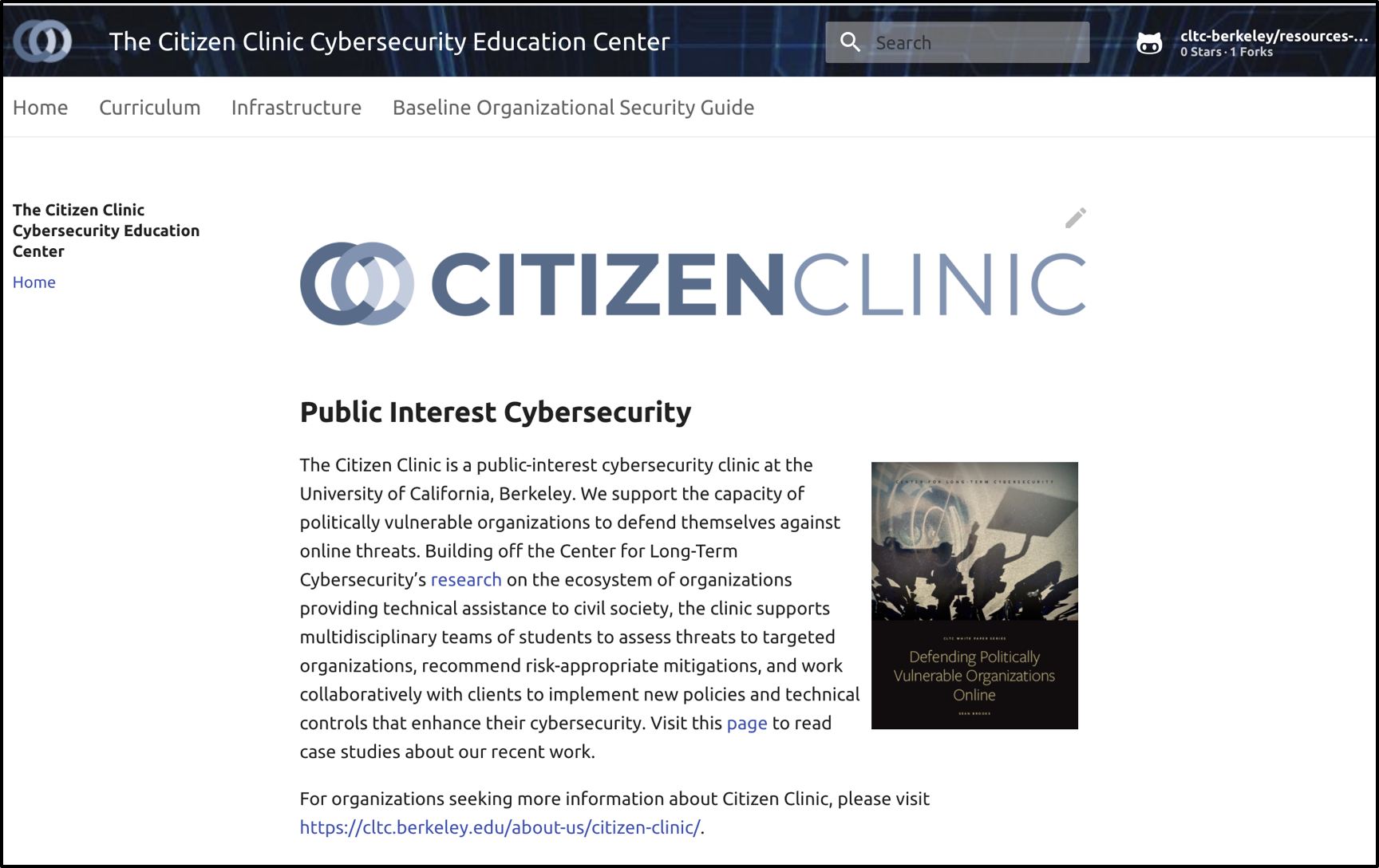The image is a horizontally-oriented rectangle bordered by a thin black line. At the top of the image, a dark blue banner spans from left to right. On the far left of this banner, there are two overlapping circles in a light blue or grayish hue. Within the banner, in white text beginning closer to the left, it reads "Citizen Clinic Cybersecurity Education Center."

Just past the center of the banner on the right side, there is a gray search box with a search icon. Further to the right is a small emblem featuring a raccoon, accompanied by tiny, hard-to-read text.

The main section of the image has a white background. At the top, aligned to the left, the text reads "Home Curriculum Infrastructure Baseline Organizational Security Guide." This text is underlined by a very thin gray line.

In the upper left within this main section, it says "Citizen Clinic Cybersecurity Education Center Home." Centrally located are the two overlapping circles from the banner, again in light bluish-gray. Below these circles, "Citizen Clinic" is written in bold grayish-blue text.